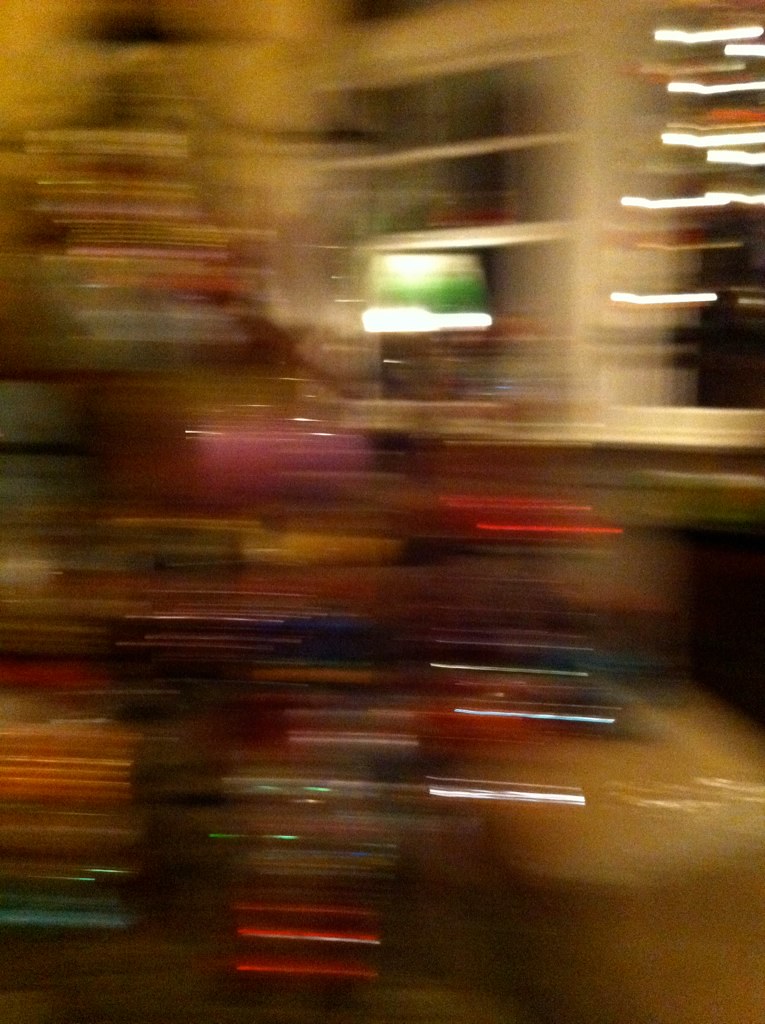This extremely blurry photograph appears to have been taken indoors while the camera was in motion, perhaps moving from left to right. The setting resembles a bookstore, with numerous books stacked vertically from floor to ceiling, creating colorful streaks of red, blue, orange, yellow, pink, and purple across the image. In the background, higher up, you can discern at least two windows that indicate it is nighttime outside, characterized by streaky lights. An emerald green lampshade sits atop a table lamp, adding a touch of ambient light to the scene. The walls, painted in an off-white hue, provide a subtle backdrop to the vibrant and somewhat chaotic visual elements.